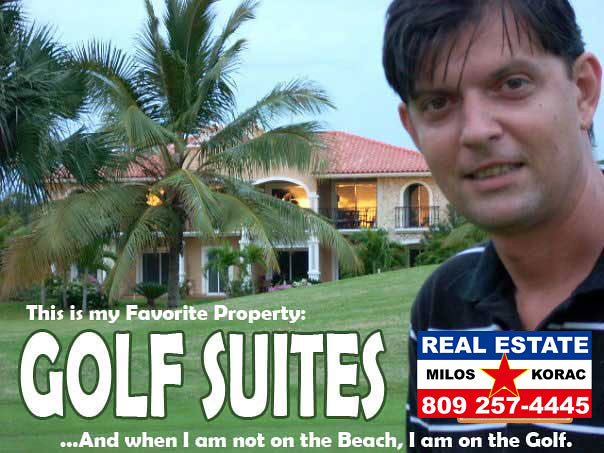This is an advertisement for a real estate agent named Miloš Korak. Set against a backdrop of lush greenery with a sloping hill, palm trees, and a stunning, large beachfront property, we see Miloš Korak standing on a well-maintained lawn. The property features a distinctive red roof and red-orange walls with white-bordered windows and doors, under a clear blue sky.

In the upper right-hand corner of the ad is a close-up picture of Miloš's face. He is in his 40s with brown hair, bangs, a clean-shaven face, and a fair complexion, smiling directly at the camera. He is wearing a blue and white striped shirt.

Overlaying his shirt in the bottom right is a logo consisting of three horizontal bars: blue, white, and red. The red bar features a central red star with the white text "Real Estate," and the white bar has "Miloš Korak" written in black text. The bottom red bar has his phone number, 809-257-4445, in white text.

To the left of the logo, the ad reads: "This is my favorite property, Gulf Suites. When I'm not on the beach, I am on the golf." This text suggests that the property might be part of a golf course, further highlighting its prime location and appeal.